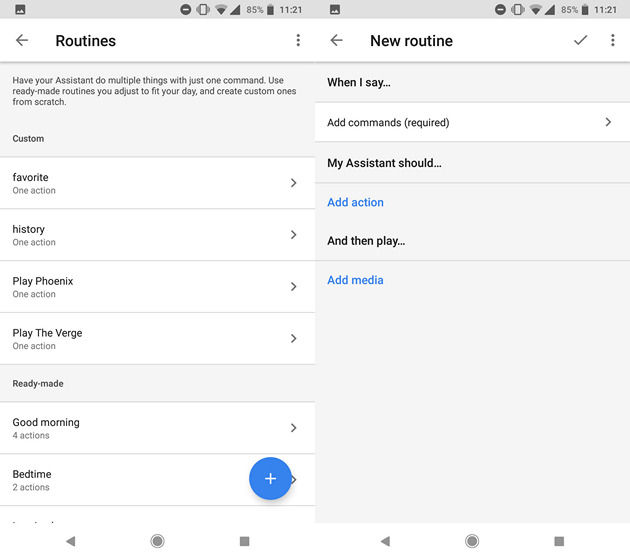### Website Interface Screenshot Description

**Header Bar:**
- **Color**: Grey
- **Icons**: 
  - **Photographs** with a **minus sign** next to it
  - **Vibration** indicator
  - **Wi-Fi** signal (not at full strength)
  - **Battery** level at **85%**
- **Time**: Displayed as **11:21**

**Main Screen:**
- **Two Identical Sections** side-by-side, each displaying the same time and items.

**Left Section**:
- **Header**: "Routines: Have your assistant do multiple things with just one command."
  - **Tagline**: "Use ready-made routines you adjust to fit your day and create custom ones."
- **Custom Routines**:
  - **Favorite One Action**
  - **History One Action**
  - **Play Phoenix One Action**
  - **Play The Verge One Action**
- **Ready-Made Routines**:
  - **Good Morning**: 4 actions
  - **Bedtime**: 2 actions
- **Add More**: Indicated by a **plus sign**

**Right Section**:
- **Header**: "New Routine"
  - **Tagline**: "When I say"
- **Commands**:
  - **Add Commands**: (required)
  - **Add Action**
  - **Add Media**

This detailed caption captures the layout and functionalities depicted in the screenshot effectively.